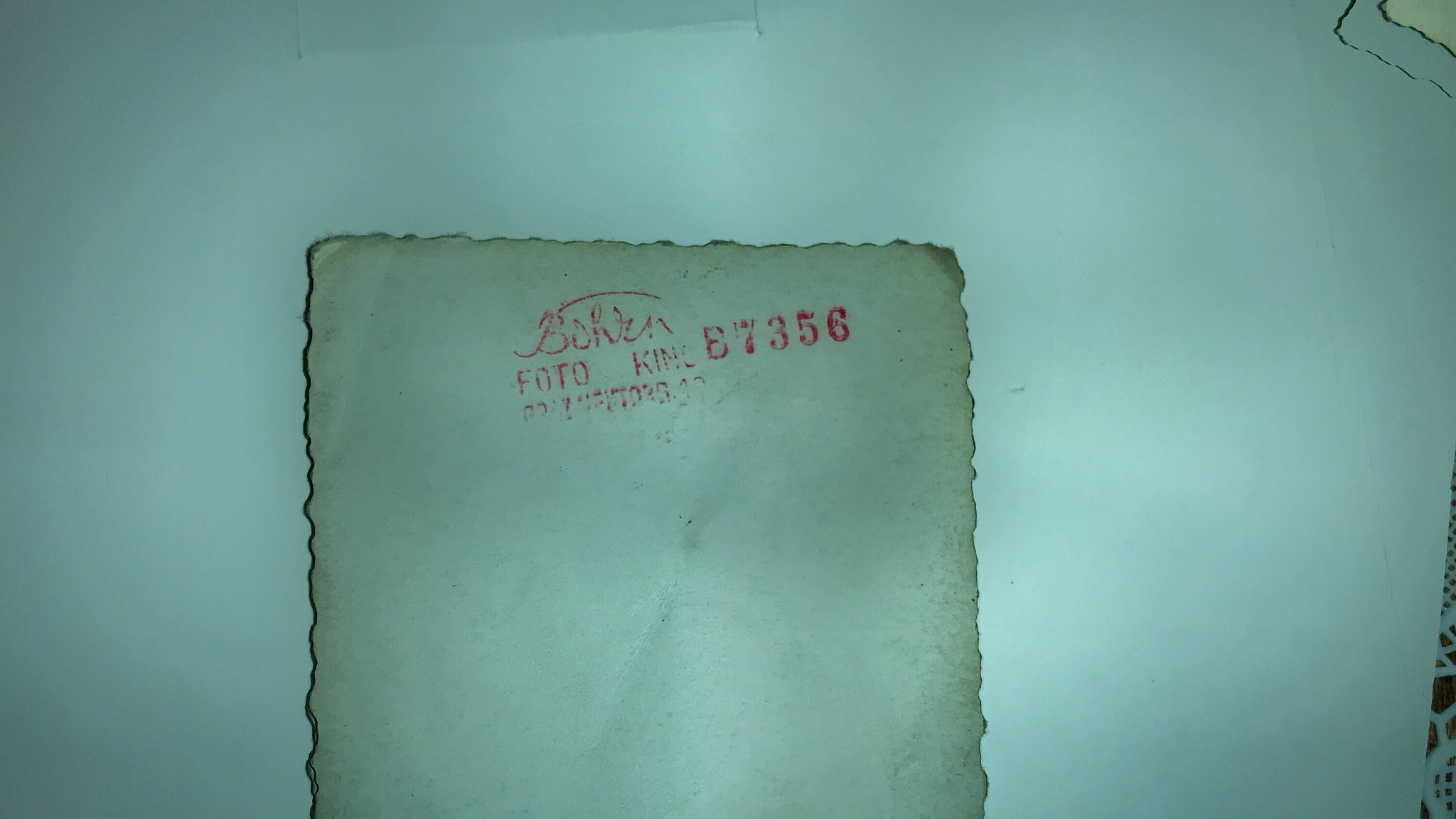The rectangular image captures an overhead view of a table or countertop illuminated by a fluorescent light, creating a blend of blues and light blue hues. Centered on the countertop is the back of a vintage photograph, characteristic of early 1900s prints with slightly irregular, darker black edges. The aged white back of the photograph features red stamped text at the top, clearly stating "BOWERN FOTO KING," with 'FOTO' spelled in an old-fashioned manner. Additionally, a red ink number "87356" is prominently displayed, adding to the authentic vintage appearance of the image.